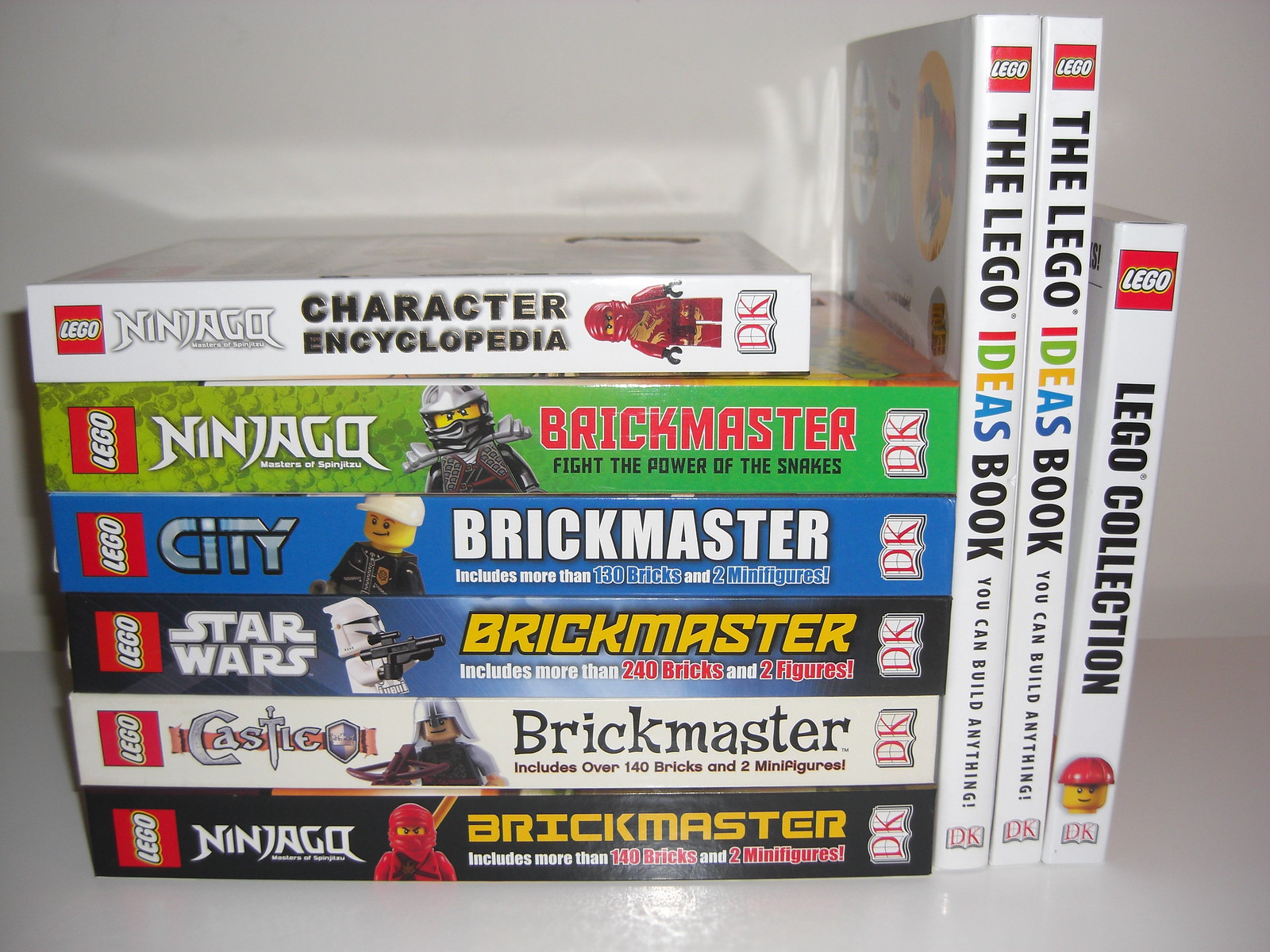The image displays an assortment of nine LEGO-themed books neatly arranged on what appears to be a white surface against a white background. Six books are stacked horizontally, with the titles clearly visible. From top to bottom, the books are: "LEGO Ninjago Character Encyclopedia," showing a LEGO ninja on the cover; "LEGO Ninjago Brickmaster: Fight the Power of Snakes," featuring a LEGO figure in a black and gray outfit on a green background; "LEGO City Brickmaster," which includes more than 130 bricks and two minifigures; "LEGO Star Wars Brickmaster," which contains over 240 bricks and two minifigures; "LEGO Castle Brickmaster," with a knight illustration, offering more than 140 bricks and two minifigures; and another "LEGO Ninjago Brickmaster," also including over 140 bricks and two minifigures. Standing vertically beside these are three additional books: the first two are "LEGO Ideas: You Can Build Anything," and the last one is "LEGO Collection," which features a LEGO figure with a red helmet on the cover.